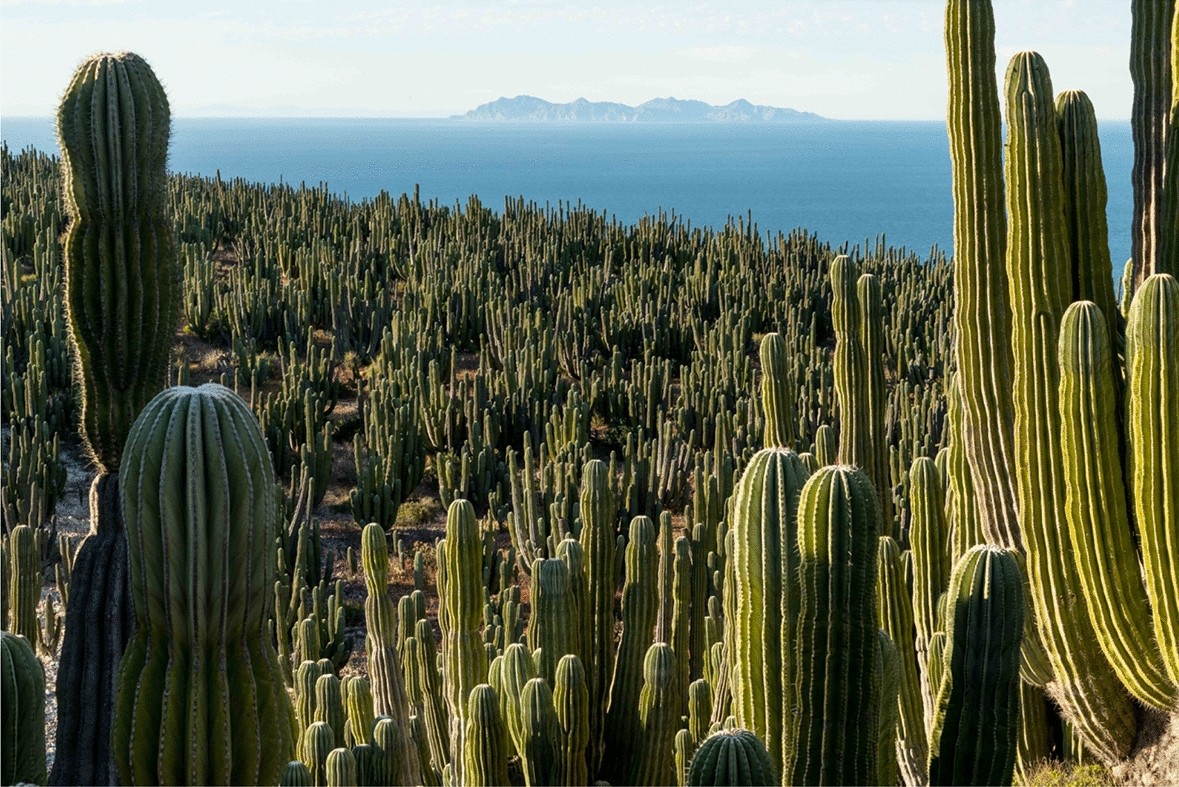This detailed color photograph, presented in landscape orientation, showcases an expansive desert scene filled with hundreds, possibly thousands, of cacti. Dominating the foreground are towering cacti, standing about 8-9 feet tall with multiple green sprouts. The cacti field stretches across the bottom two-thirds of the image, presenting a seemingly endless sea of prickly vegetation. The desert floor is punctuated by patches of dirt and sparse grass. Toward the top third of the image, a blue body of water or what appears to be an ocean, blends confusingly with the desert scene. This causes a surreal and puzzling effect, further accentuated by a small, hazy, grayish mountainous range perched on the distant horizon. The sky above has a hazy, whitish-gray tint. The photograph embodies a blend of realism and photographic manipulation, as the superimposition creates an intriguing juxtaposition of desert and ocean elements, leaving the viewer to ponder the extraordinary composition.